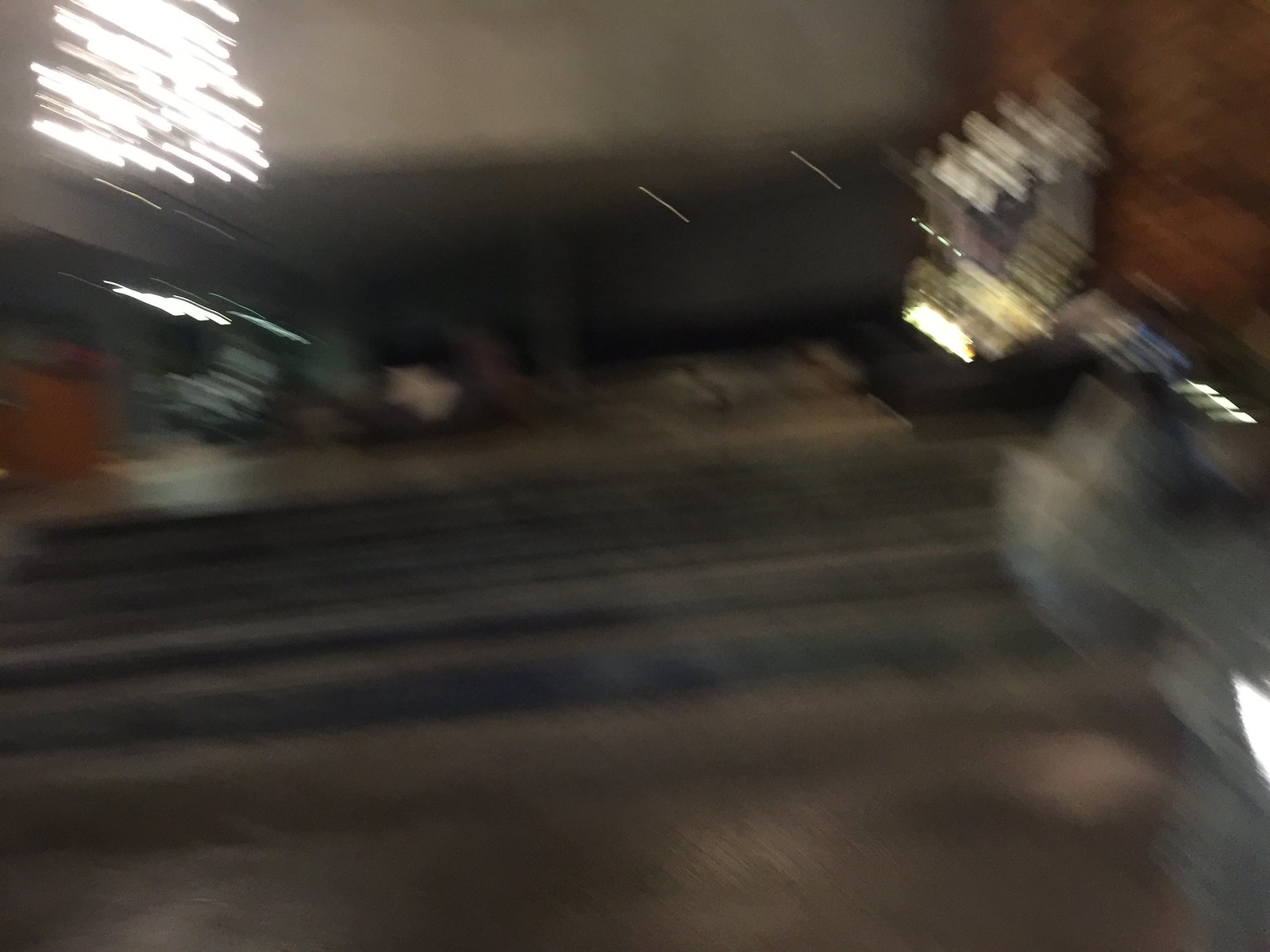An indistinct, blurry image is depicted with various elements scattered throughout the frame. In the top left corner, a series of bright, short vertical lines are grouped together, appearing somewhat like streaks of light. The upper portion of the image features a horizontal area with a tan coloration. In the top right corner, a hint of red is visible, accompanied by a reflective surface nearby that catches some light. Additional bright vertical lines can be seen along the right edge. The background, situated below the tan horizontal strip, is shrouded in darkness, with possibly a few posts faintly discernible. The ground features predominantly brown hues, marked by black horizontal lines running across its surface.